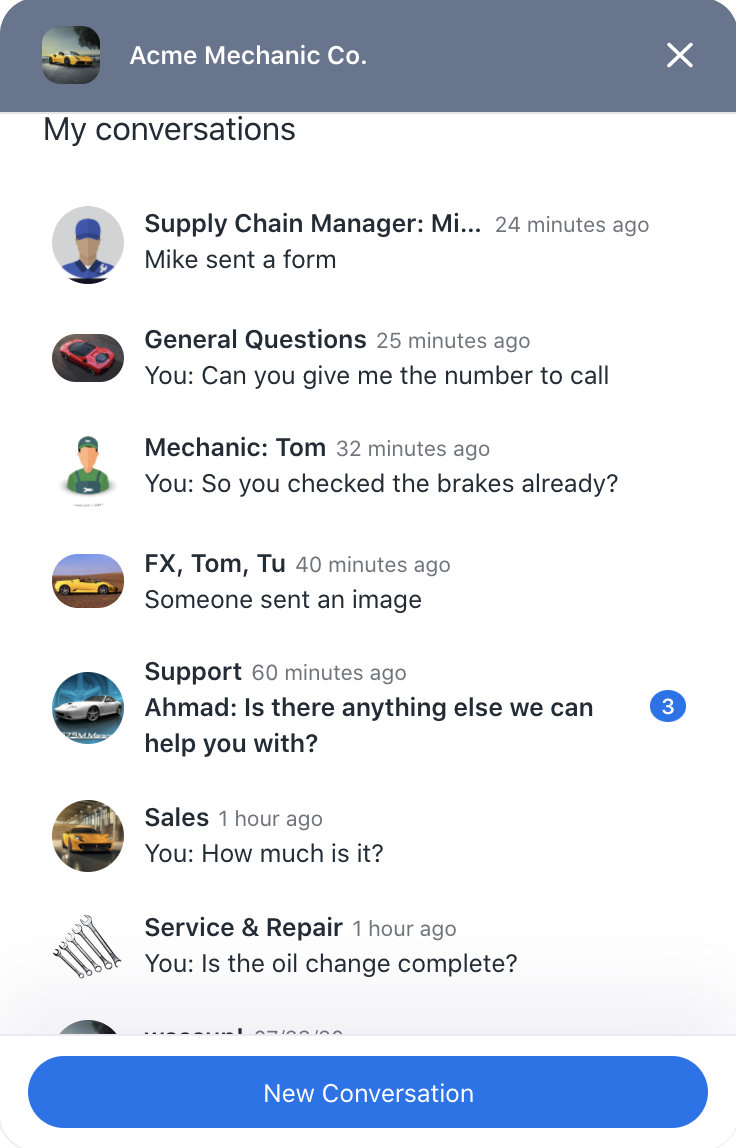The image appears to showcase a detailed view of a comment or chat section on a website. At the very top of the page, there's a thick, light gray bar running horizontally across the entire width. On the left side of this bar is a somewhat square, colored picture with rounded edges, depicting a yellow card aligned beside a tree. To the right of this image, in white text, it reads "Acme Mechanic Co." followed by a period. Farther to the right within the bar is a white "X."

Beneath this gray bar, the background turns white, with all text presented in black. In the top left corner, it reads "My Conversations." Directly below this text is a gray circle avatar, featuring a faceless man donning a blue ball cap and jacket. Adjacent to this avatar, it states "Supply Chain Manager, MI" with an ellipsis following and "24 minutes ago" to the right. Below this, it notes, "Mike sent a form."

Further down, an oblong circular image shows a red car. Next to it, the text reads, "General Questions, 25 minutes ago." Below this line, it says, "You: Can you give me the number to call?"

Continuing downward, there is a right-facing circle depicting a faceless man in a green visor, T-shirt, and apron. Next to this avatar, the text reads, "Mechanic: Tom, 32 minutes ago." Below this, it says, "You: So you checked the brakes already?"

Beneath this, another elongated circular image displays a yellow car in the desert facing to the right. Adjacent to this picture are the letters "FX," followed by "Tom, T-U, 40 minutes ago." Below this line, it indicates that someone sent an image.

Further down, a circle contains a gray car against a blue background. Next to it, the text reads, "Support, 60 minutes ago," and underneath, it says, "Ahmed, R: Is there anything else we can help you with?" To the right is a blue circle with a white numeral 3 inside.

Continuing, another circle shows a gray car in front of a building. Next to it, it states, "Sales, one hour ago." Below this, "You: How much is it?"

Farther down, another image of five wrenches, slightly angled and lined up from left to right, appears with the text "Service & Repair, one hour ago." Below this line, "You: Is the oil change complete?"

Finally, at the bottom of the page, a long blue bar is visible. Inside this bar, in white text, it states, "New Conversation."